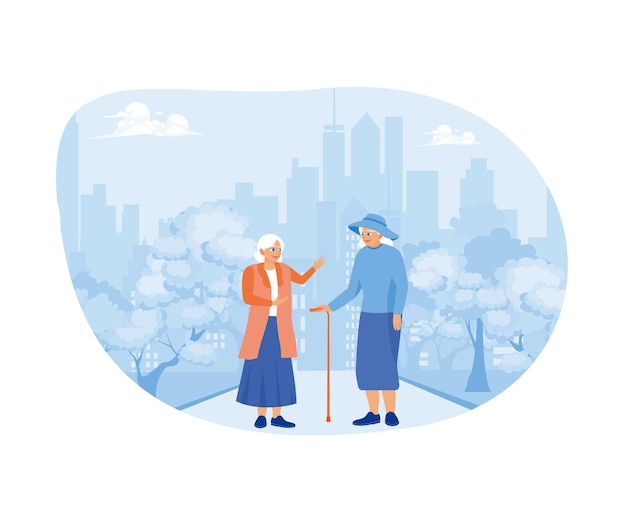This is a detailed cartoon illustration set within a blue-toned, bubble-like, oval-shaped structure on a white background. At the center of the circular artwork, a pathway spans horizontally where two elderly cartoon characters stand engaged in conversation. On the left side of the path is a shorter woman wearing a red jacket over a white shirt, paired with a large blue skirt and blue shoes. Her hair is gray. On the right side, there is a taller woman, also with gray hair, dressed in a light blue shirt, a dark blue skirt, blue shoes, and a blue hat. She is holding a cane in one hand. The surroundings feature blue-shaded trees and clouds, with a backdrop of tall skyscraper buildings, evoking a cityscape atmosphere. The serene scene is nested within a smooth, non-uniform circular boundary, giving it a whimsical and contained feel.